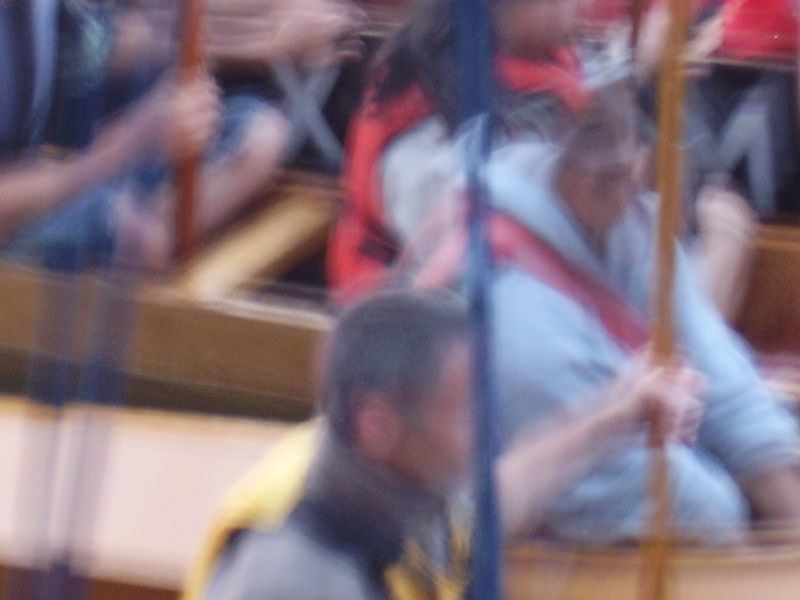This blurry image captures the interior of what appears to be a boat, with several people holding onto ropes or bars for support. In the foreground, there is a man wearing a yellow life vest. Behind him, towards the right side of the image, a person with long hair, likely a woman, is visible wearing a coral-colored life vest.